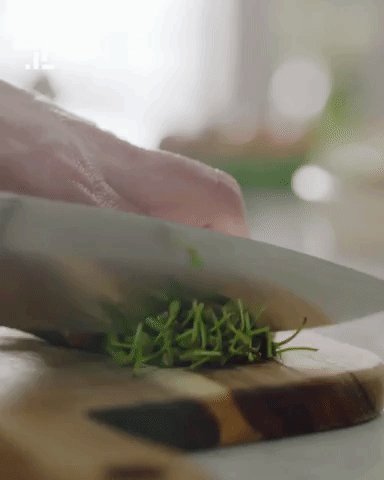The image is a blurry close-up shot of a person chopping green vegetables on a wooden cutting board. Despite the poor focus, the wood grain and varying colors of the board are distinctly visible, suggesting a soft texture. A large silver butcher knife is in use, and a white hand, likely from an older individual given the description of wrinkles, is holding down the vegetables, implying it’s the left hand. The scene appears to be set on a white table in a brightly lit kitchen. Although the background is indistinct, there are hints of orange and green elements, possibly other kitchen items or décor.